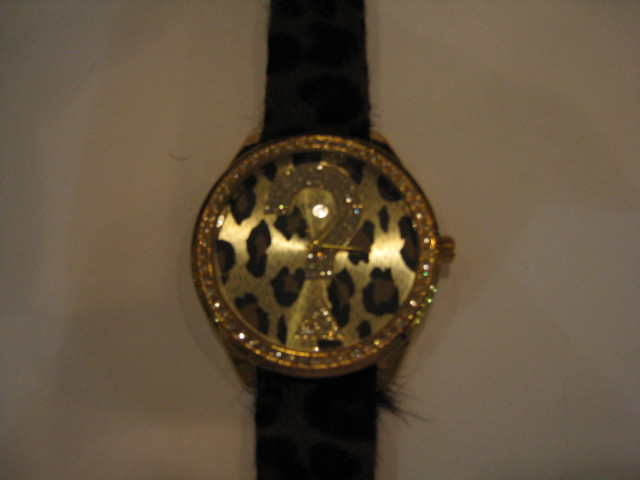This low-resolution, poorly-taken landscape photograph captures a close-up of an extremely ugly wristwatch positioned on a white surface. The dark tan background is shadowy, adding to the image's ineffective detail. The watch features a frayed, almost hairy-looking black band that wraps around the wrist. The circular watch face, obscured by shadows and blurriness, has a goldish border adorned with sparkles, resembling diamonds, but their authenticity is questionable due to their low-quality appearance. The centerpiece of the watch face is an oversized question mark, studded with more glittering elements and filled with a brown center, against a cheetah print pattern made from a slightly brassy, yellow metal. The hour and minute hands are faintly visible but can't be clearly distinguished. The watch notably lacks any numbers, which adds to its peculiar and unattractive design.